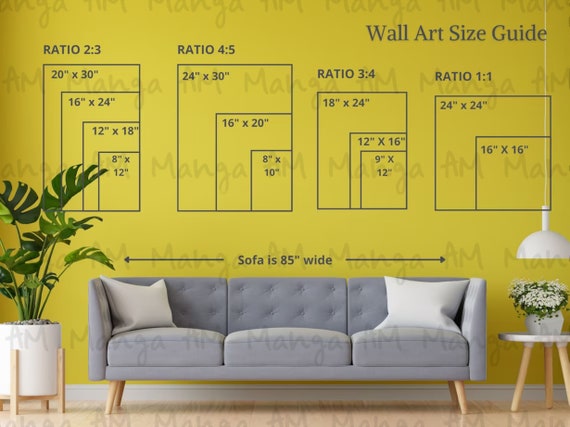In this image, there is a stylish living room centered around a gray sofa with two pillows at each end, supported by brown wooden legs. The sofa measures 85 inches wide, as indicated by the measurements displayed on top. To the right of the sofa, a white hanging lamp descends from the ceiling over a flower vase placed on a stool. On the left side, a green leafy plant resides in a white pot on a brown platform. The background features a yellow wall, albeit a somewhat dull shade, adorned with dark gray text that reads "Wall Art Size Guide." This guide includes various ratios such as 2:3, 4:5, 3:4, and 1:1, along with dimensions ranging from 8x12 inches to 20x30 inches. The entire picture illustrates the wall directly behind the sofa, filled with these size and ratio diagrams, and the colors present include yellow, gray, green, dark green, tan, and brown.